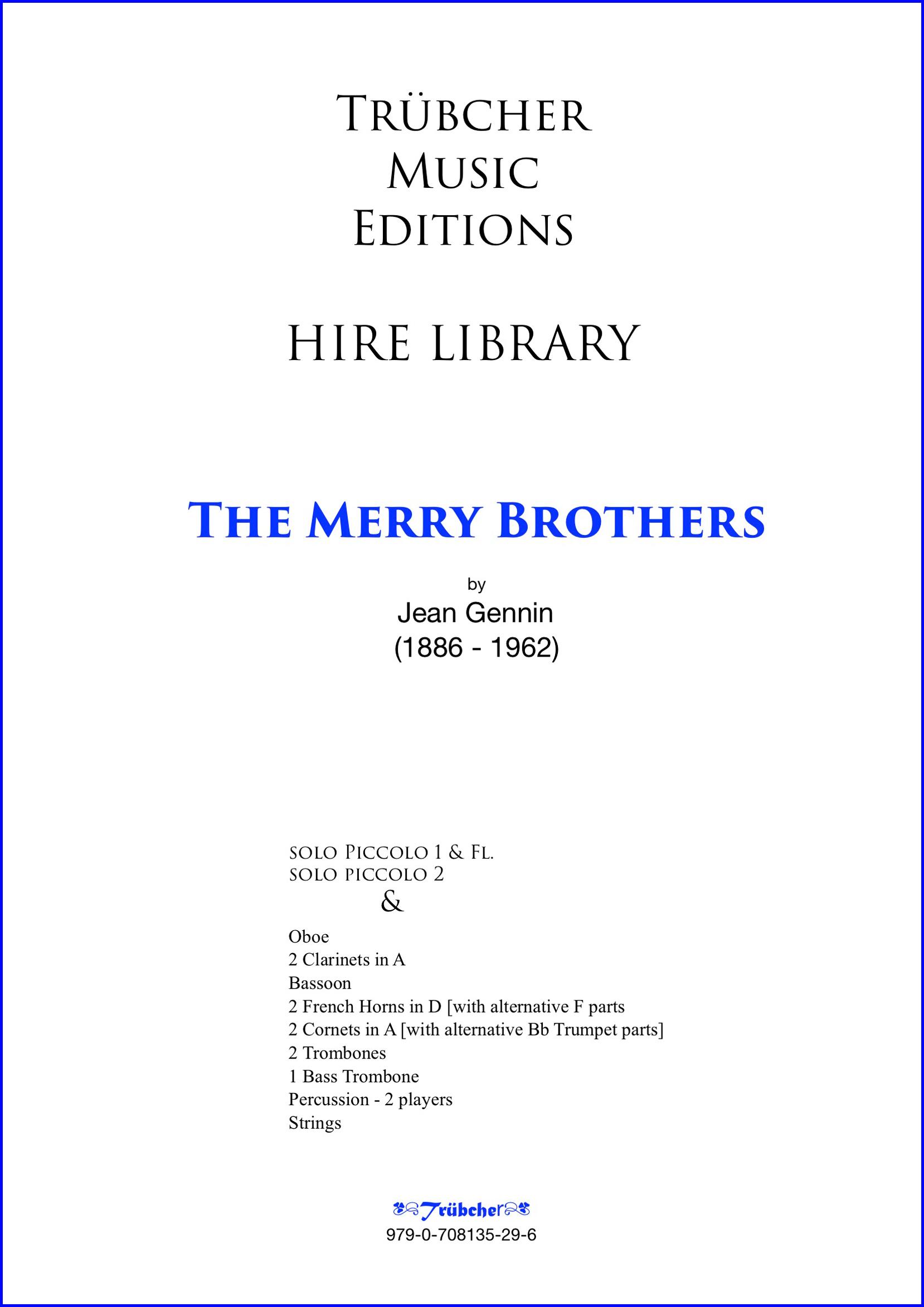The image is a detailed scanned page from a book, framed by a blue rectangular border. At the top center, in black text, it reads "Troubature Music Editions, Higher Library." Below this, in large, bold blue letters, it says "The Merry Brothers." Continuing downward in black text, it states "By Gene Ginnin (1886-1962)." Further down, the instrumentation details are listed meticulously: "Solo Piccolo I and FL, Solo Piccolo II, Oboe, two Clarinets in A, Bassoon, two French Horns in D (with alternative F parts), two Cornets in A (with alternative Bb Trumpet parts), two Trombones, one Bass Trombone, Percussion (two players), and Strings." Near the bottom, there is blue text in a foreign language that seems to include the word "Troubature" again, followed by what appears to be a catalog number in black text: "979-0-708135-29-6." The background of the page is white.